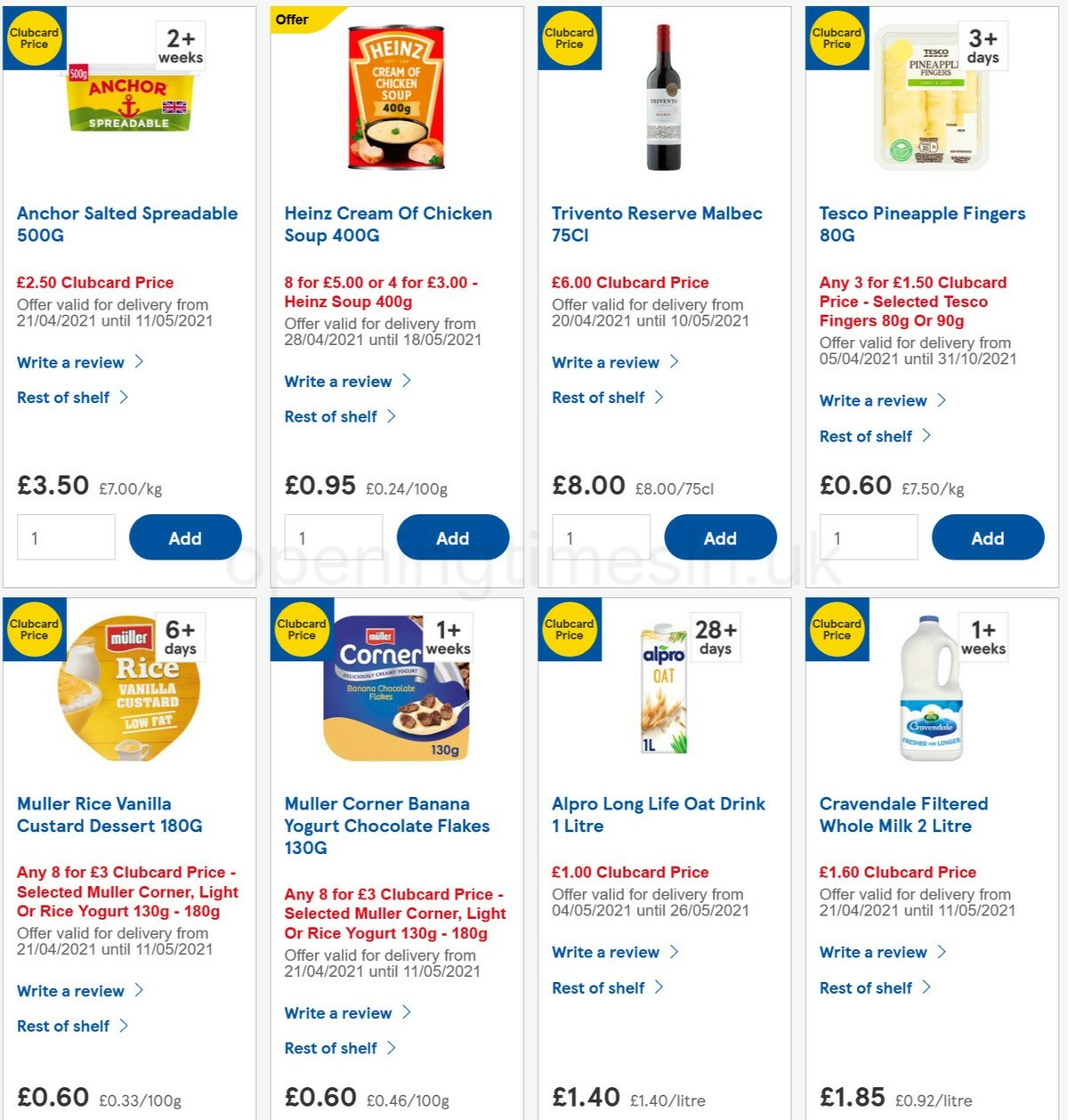This screenshot showcases an online grocery catalog with a white background, featuring a neat arrangement of product listings in a grid format. There are two rows, each containing four vertical rectangles, making a total of eight product listings.

Each rectangle follows a uniform layout:
- At the top center is an image of the grocery item.
- Below the image, the item's name is displayed in blue text.
- Further down, the price of the item is highlighted in red.
- Beneath the price, there are about two lines of gray text indicating the offer validity period.
- Following this, there are two interactive links in blue text: "Write a review" and "Rest of shelf," each accompanied by a right-pointing gray arrow that resembles a sideways V.
- At the bottom left of each rectangle, the price of the item is repeated.
- Directly underneath the price, there is a light gray-outlined rectangle showing the quantity.
- Adjacent to the quantity box is a blue oval "Add" button, with "Add" written in white text.

In the bottom row, the listings are cut off at the price section, hence the quantity box and "Add" button are not visible.

The products displayed include a variety of grocery items such as butter, chicken soup, wine, and milk.